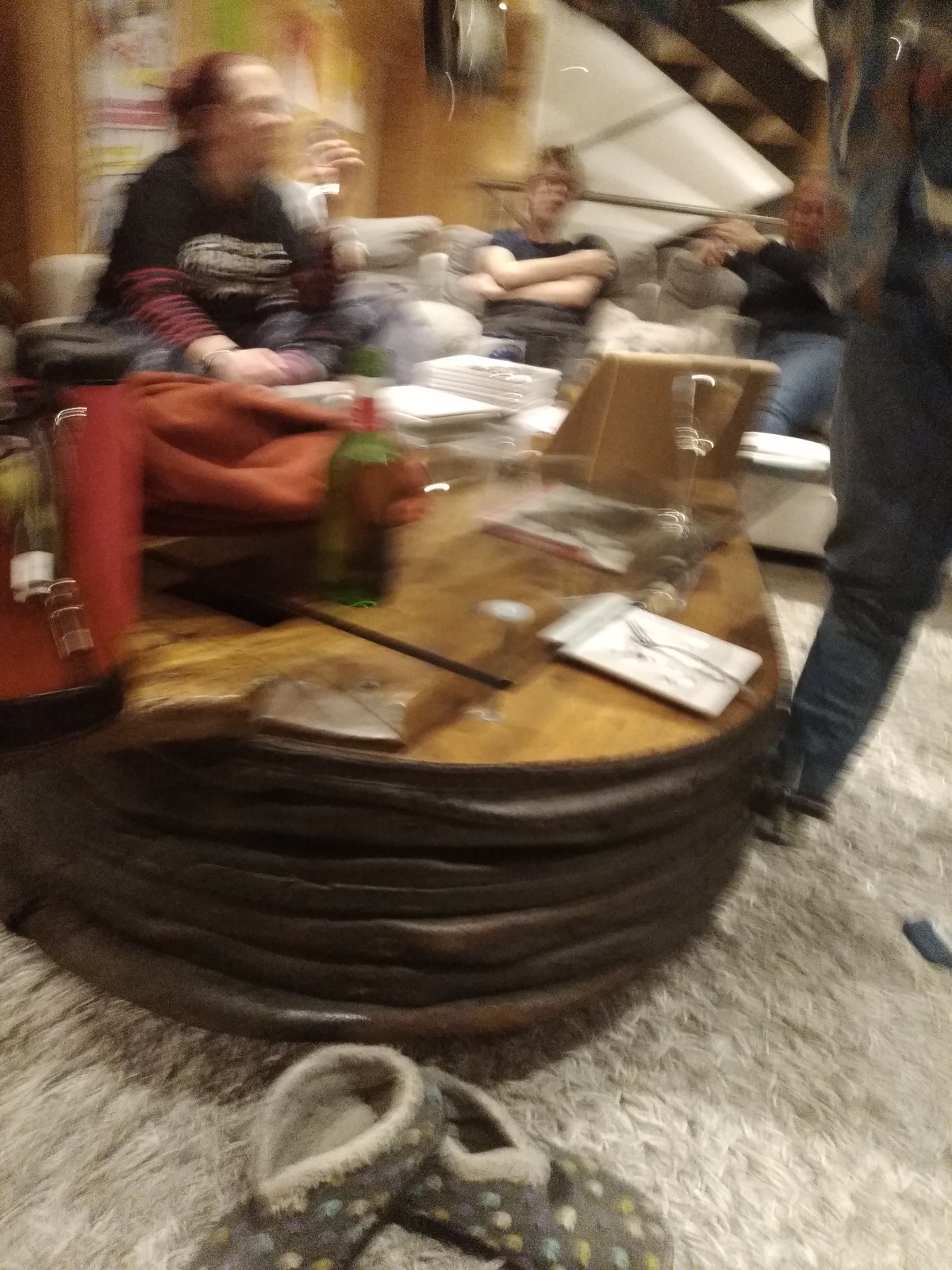In this extremely blurry image, a group of teenagers is gathered around a wooden table, sitting on what appears to be a sectional white couch. The couch extends in both directions, with two people visible on it and another person, seemingly a female, seated to the left wearing an orange jacket draped over the table. The wooden table in front of them holds a bottle, which appears to be liquor, and a notepad. In the foreground, there are a pair of gray slippers with blue, yellow, and white polka dots, seemingly placed at random. The floor features a whitish, feathery-textured carpet. To the right of the image, a person is standing, but their face and neck are completely cut off from the frame, adding to the disjointed feel of the photograph. The image's extreme blurriness makes it difficult to discern any further details, raising the question of whether the blur was intentional or a result of an unfocused shot.